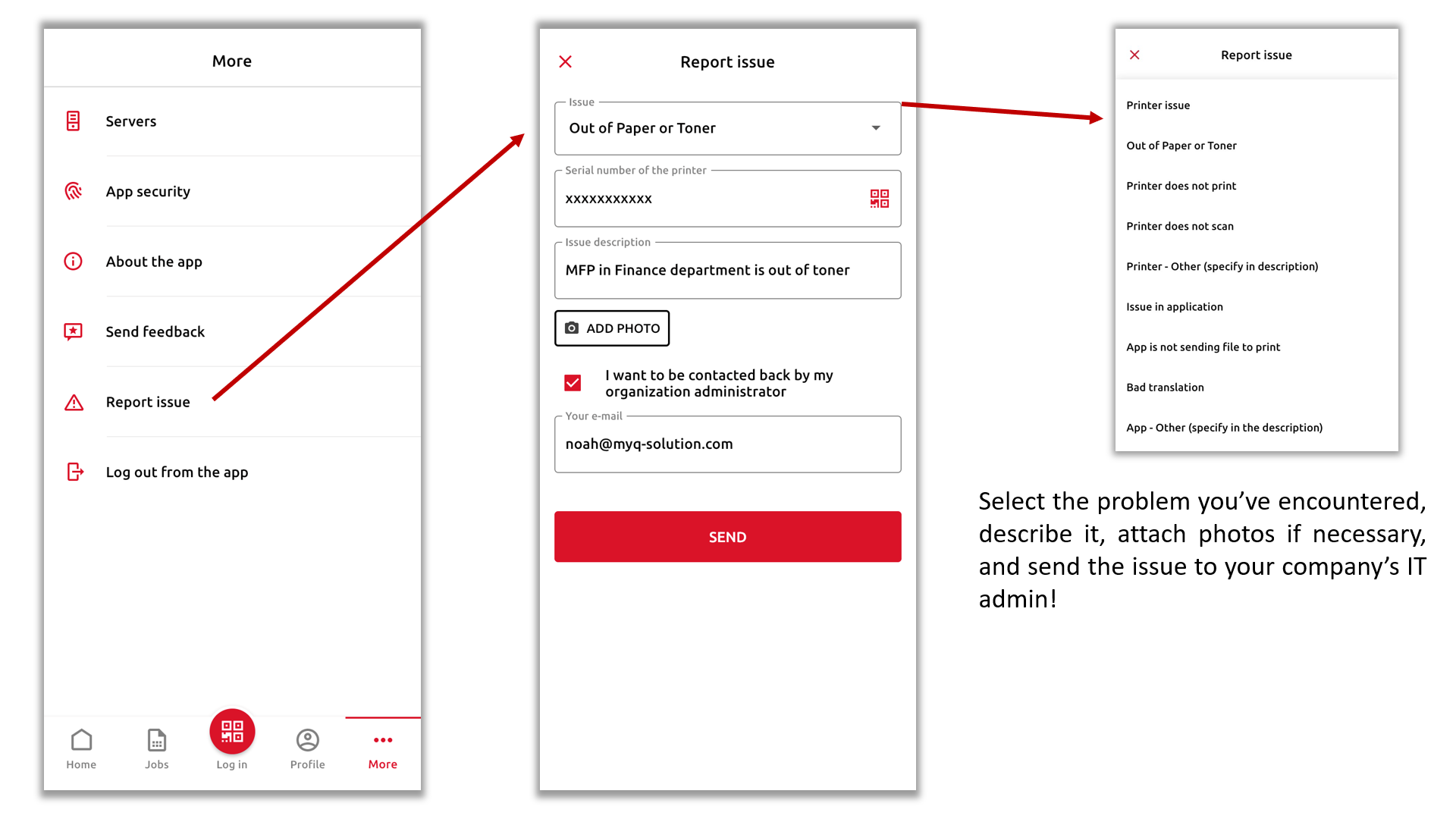This image collage consists of three consecutive phone screenshots, arranged from left to right, with arrows indicating the sequence of actions. The left screenshot displays a menu of options including "Servers," "App Security," "About the App," "Send Feedback," "Report Issue," and "Log Out." A red arrow points from the "Report Issue" option to the middle screenshot. 

The middle screenshot shows a drop-down menu titled "Report an Issue," where "Out-of-Paper/Toner" is selected. From this selection, another red arrow points to the third screenshot.

The right screenshot highlights a form where the issue is specified as "Printer Issue: Out-of-Paper/Toner." This comprehensive visual guide instructs users on how to navigate the app to report a printer issue due to being out of paper or toner.